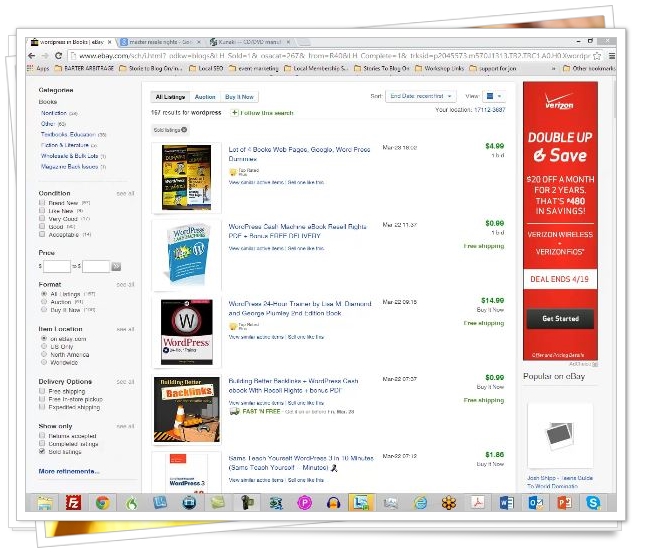A slightly blurry screenshot captures the search results page from eBay.com. On the left-hand side, a grey panel displays various filters such as categories including "Books & Notebooks" and "Textbooks & Education." Further options allow users to specify the condition of the item, set a price range, choose a format, determine item locations, and select delivery options. There is also an obscured element at the bottom of the panel. The search term "WordPress" yields 167 results, prominently displaying five book listings underneath. On the right-hand side of the screen is a large advertisement for Verizon, promoting a deal dubbed "Double Up and Save" which offers $20 off per month for two years, resulting in $480 in total savings. The offer ends on April 19, and there is a noticeable black button with white text prompting users to "Get Started." The visible book titles in the search results include entries related to WordPress, webpages, and Google, although some titles are partially obscured. Each listing is highlighted in blue text with respective prices listed to the right.